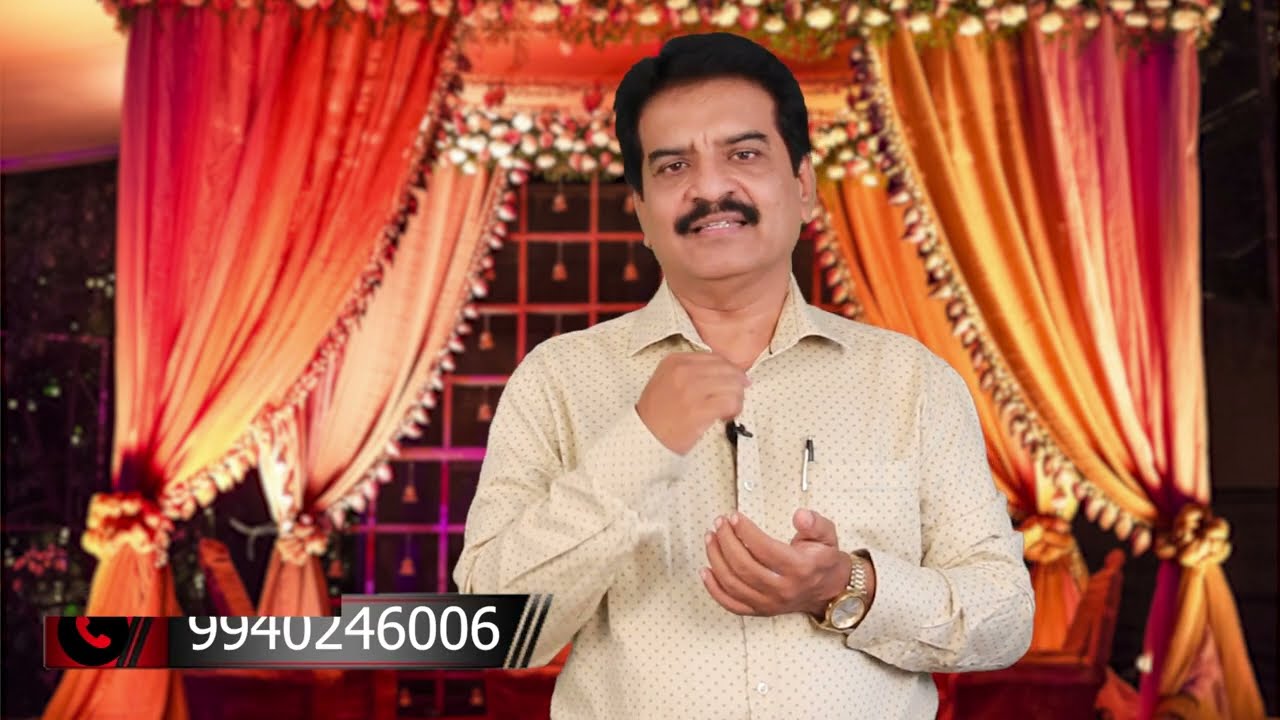The image appears to be a screen capture from a video, showing a man who seems to be of Indian descent. He is in his 40s, with dark brown hair and a matching dark brown mustache. He is staring into the camera with a serious expression. The man is dressed in a button-up shirt with a light beige or off-white color featuring a subtle checkered or polka dot pattern. A silver pen is visible in his left shirt pocket. He wears a gold wristwatch on his left wrist and has a lapel microphone clipped to his shirt.

The background behind him features a colorful, draped curtain in shades of orange, red, yellow, and pink with sequins and flashy objects. These curtains are pulled back to reveal a bed with a canopy adorned in bright, vibrant colors, contributing to a bedroom-like scene. Additionally, behind the man, there are some walls with black squares and red lines.

In the bottom left corner of the image, there is a telephone icon followed by the number 9940246006 in white font, indicating that this is likely part of a live program.